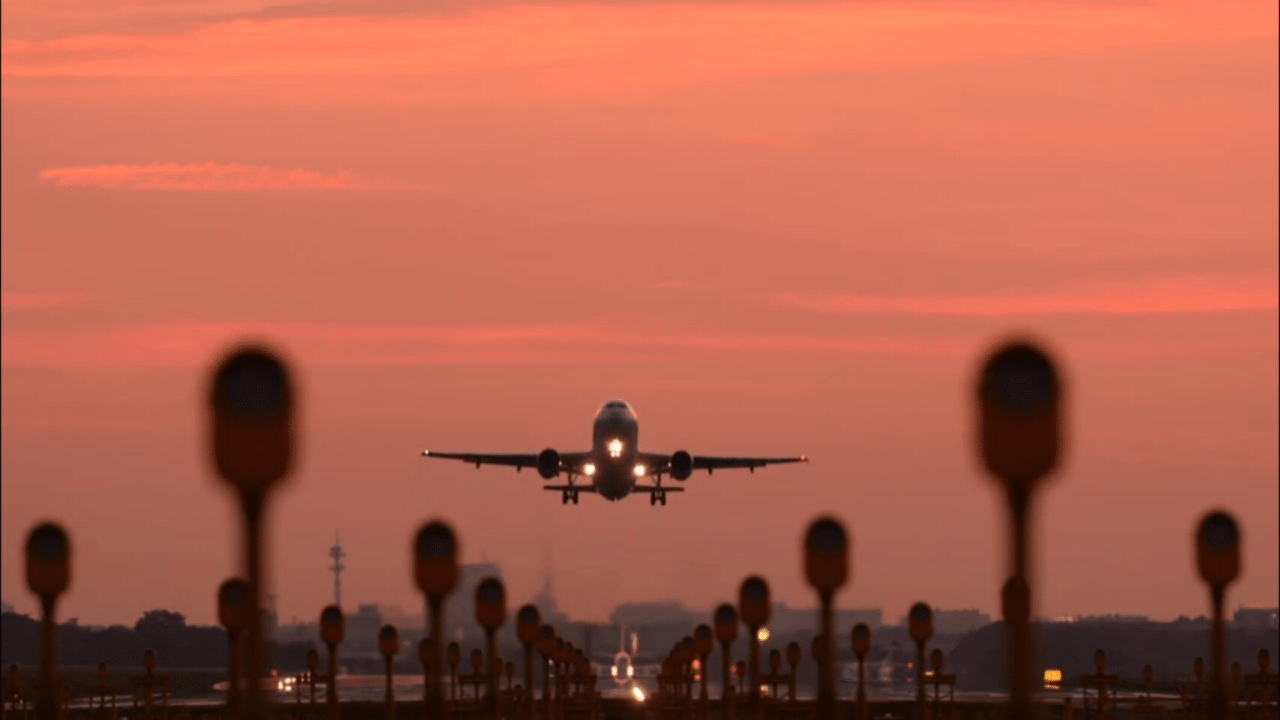In this striking image, an airplane, painted in a sleek white, is prominently featured as it ascends into the sky, having just taken off from the runway. The vantage point from below the aircraft captures its underbelly, where three bright lights and extended wheels are visible, emphasizing its rise in elevation. The background is bathed in a stunning reddish hue, evocative of either a sunset or sunrise, lending a dramatic, cotton candy-like appearance to the sky. Below the plane, the airport from which it departed is faintly discernable, along with blurry warning posts and traffic cones that mark the area. Additionally, in the far distance, another plane can be seen preparing for takeoff, with airport towers and dimly lit buildings or hills adding depth to the backdrop. The image masterfully captures the dynamic beauty of aviation against a rich, atmospheric sky.